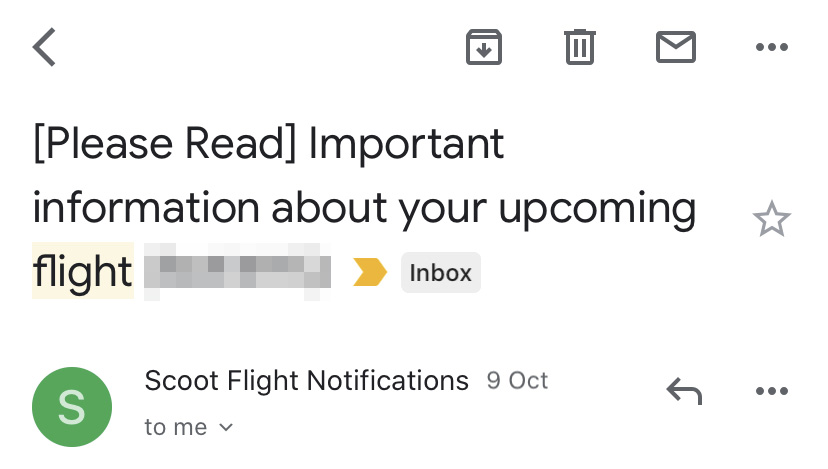The image is a screenshot of an email notification with a white background. At the top left corner, there is a dark green back button in the shape of a left-facing caret. To the right of this button, a series of icons are visible, including a download icon, a trash bin, and an envelope icon, presumably for saving, deleting, and managing the email, respectively.

The email is from "scoot flight notifications" and was sent on October 9th. The subject of the email, prominently displayed, reads "Please read: Important information about your upcoming flight." To the left of the subject line, a green circular icon with an uppercase gray "S" is visible. Directly beneath the subject line, the recipient field indicates the email was sent to "me," accompanied by a down-facing arrow caret.

The body of the email is partially blurred, obscured by a gray pixelation, making the details unreadable. On the right side of the email body, there is a curved arrow icon, likely intended for forwarding the message.